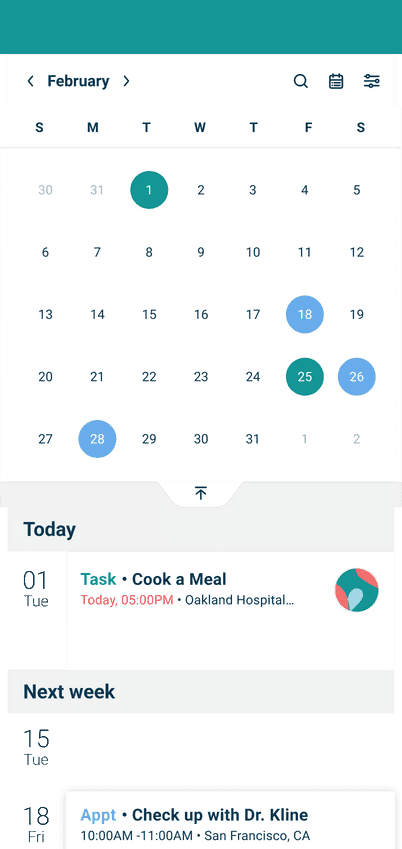The image displays a digital calendar from an application, showcasing the month of February, incorrectly listing 31 days. Certain dates are highlighted in mild warm or neutral colors. Specifically, the 1st and 25th are circled in green, while the 18th, 26th, and 28th— a Monday— are marked with light blue circles. Various adjustable settings are available in the top-right corner of the screen.

Beneath the calendar, there is an overview of the highlighted dates. The entry for the 1st mentions a task to "Cook a meal today at 5 p.m. at Oakland Hospital" with "today" and "5 p.m." emphasized in red, and "task" highlighted in a green-teal color corresponding to the green circle on that date. Another entry notes an appointment for a check-up with Dr. Klein scheduled for February 18th, a Friday, from 10 a.m. to 11 a.m. in San Francisco, California. The term "appointment" is highlighted in light blue, matching the color of the circled date. The respective dates of these notes appear on the left-hand side of the notifications.